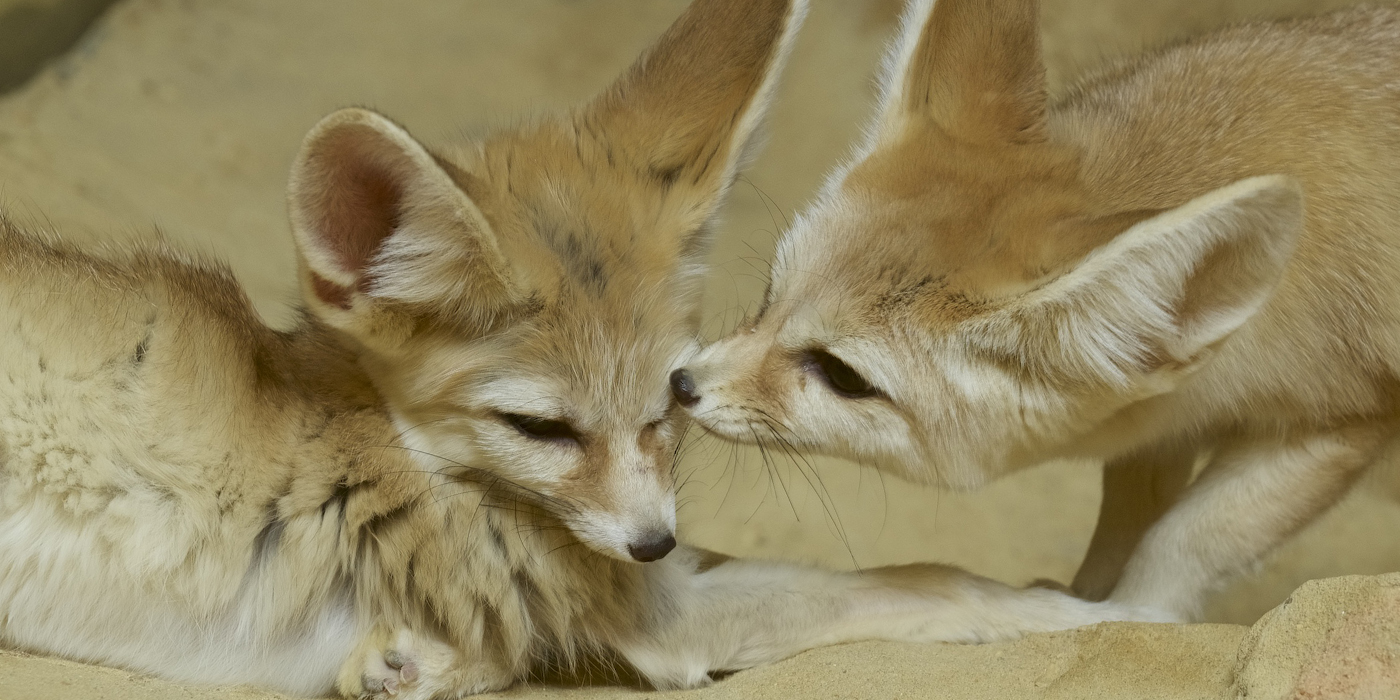This close-up photograph captures two adorable baby foxes with large, pointed snouts and very large, wide ears. The foxes have a light reddish-brown fur that transitions to white on their underbellies, with the top fur being slightly darker. Both have black eyes, black noses, and delicate whiskers. The fox on the left is lying down, facing downward, while the fox on the right is standing and sniffing the other’s head closely, almost touching it. The inside of their fuzzy pink ears is visible, adding to their cuteness. The background features a blurry, light brown, stone-like texture that complements the foxes' fur, making their delicate features stand out prominently against it.